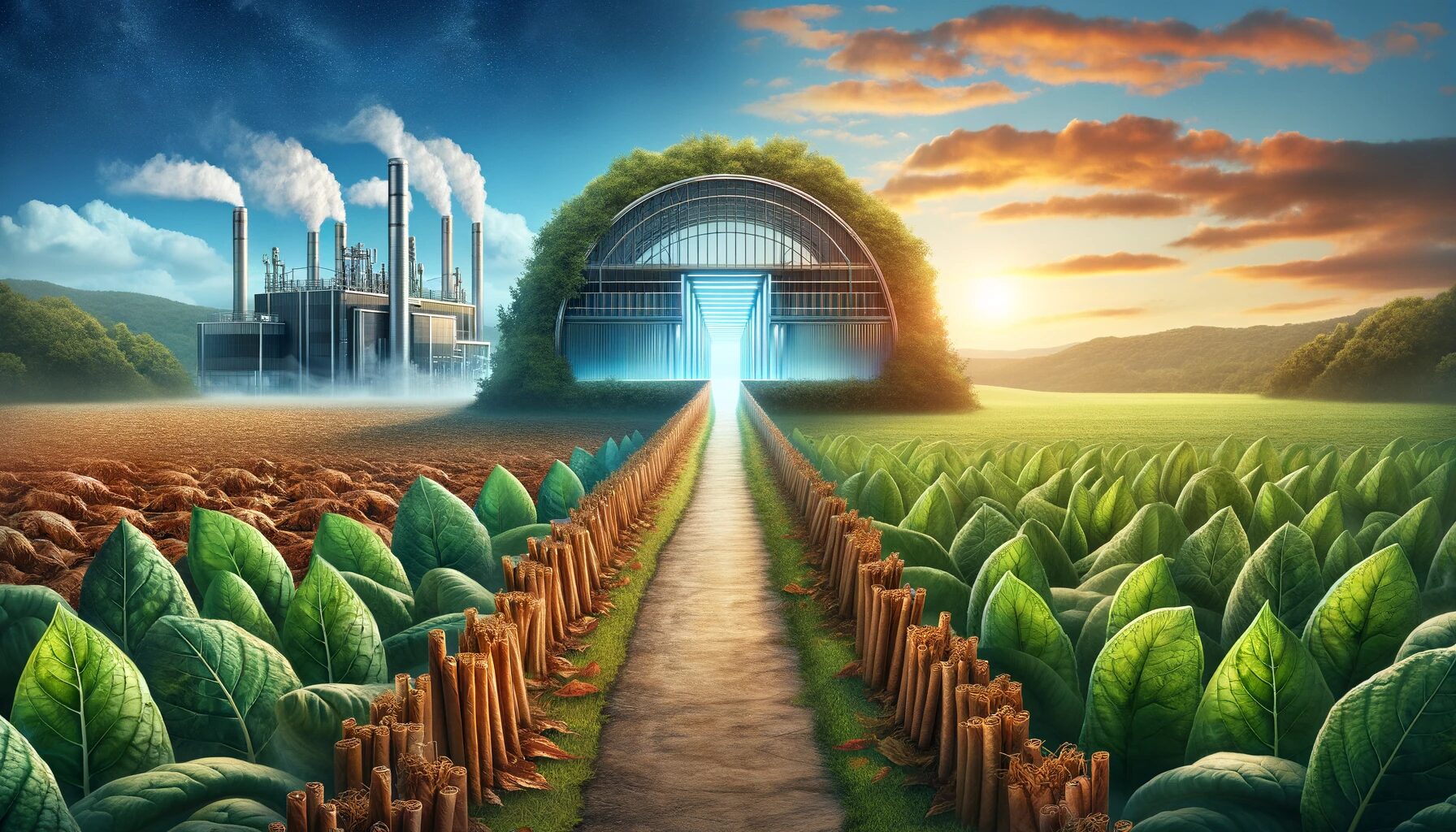The painting is a surrealist portrayal of a futuristic farming scene set outdoors, rendered in a vibrant array of colors including green, blue, brown, light green, light blue, white, and whitish gray. The image, which is a horizontally rectangular, borderless piece, features a central dirt path that stretches from the bottom center towards the top, leading to a dome-shaped building. This building is silver with vertical steel girders and is intriguingly crowned with bushy green plants, giving a sense that nature is reclaiming it. At its center is a glowing white doorway that emits a radiant light. On the right side of the path, an expansive, lush field of thick, green plants extends as far as the eye can see, under a sky adorned with beautiful, fluffy clouds illuminated by sunlight. In stark contrast, the left side of the composition showcases a factory akin to a large, silver-gray warehouse, billowing smoke into the air. This factory dominates the background with its numerous pipes and white smoke, while the foreground is marked by brown, chopped-off bamboo shoots and dead plants, underscoring a stark juxtaposition between the thriving greenery on the right and the industrial desolation on the left.